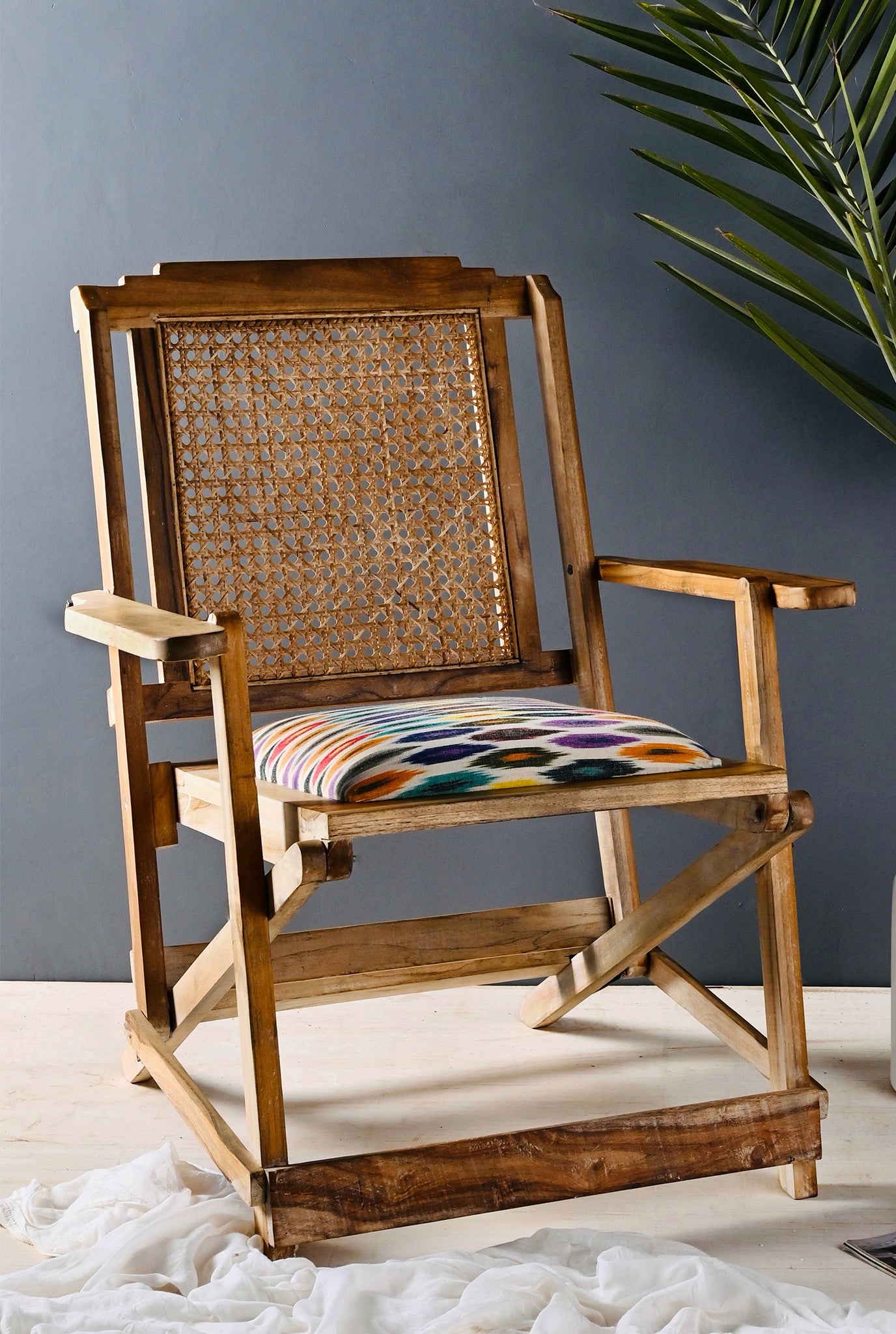The photograph captures a vintage wooden chair set against a charcoal gray-blue wall, highlighting the interior of a thoughtfully designed room. In the upper right corner, snake-like palm fronds jut out, adding a touch of greenery to the scene. The chair itself is a classic piece, characterized by its simple yet sturdy wooden structure and rattan backrest. It stands on four legs with square-shaped supports and has prominent arms. The seat features a white cushion adorned with circular designs in orange, blue, and purple, adding a modern graphic touch to the antique style. The chair is placed on a beige carpet, and the setting is completed by a bright white fabric draped on the floor, possibly a rug, which adds texture and contrast to the scene.